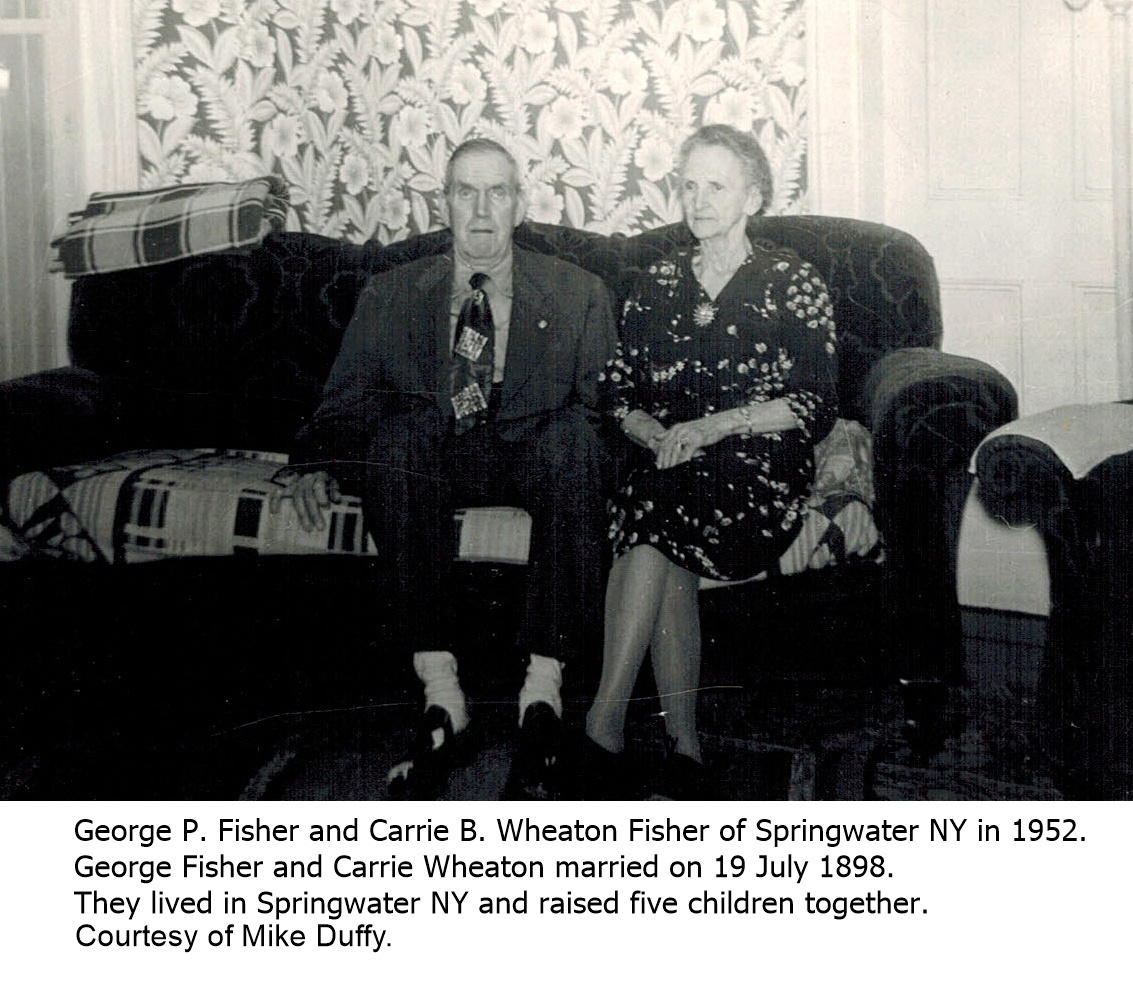This black and white photograph from 1952 captures an elderly couple, George P. Fisher and Carrie B. Wheaton Fisher, seated on a couch in their home in Springwater, New York. George, situated in the center, is dressed in a suit and tie, while Carrie, positioned to his left, dons a dress adorned with a brooch. The couch they sit on is layered with blankets—one spread across the seat cushions and another neatly folded on the back. Behind them, a floral wallpaper featuring flowers and leaves serves as the backdrop. A white panel door appears to the right of the image. The text below the photo states: "George P. Fisher and Carrie B. Wheaton Fisher of Springwater, New York, in 1952. George Fisher and Carrie Wheaton married on 19th July 1898. They lived in Springwater, New York, and raised five children together," and credits Mike Duffy. Additionally, a rug lies under their feet, complementing the cozy domestic scene.